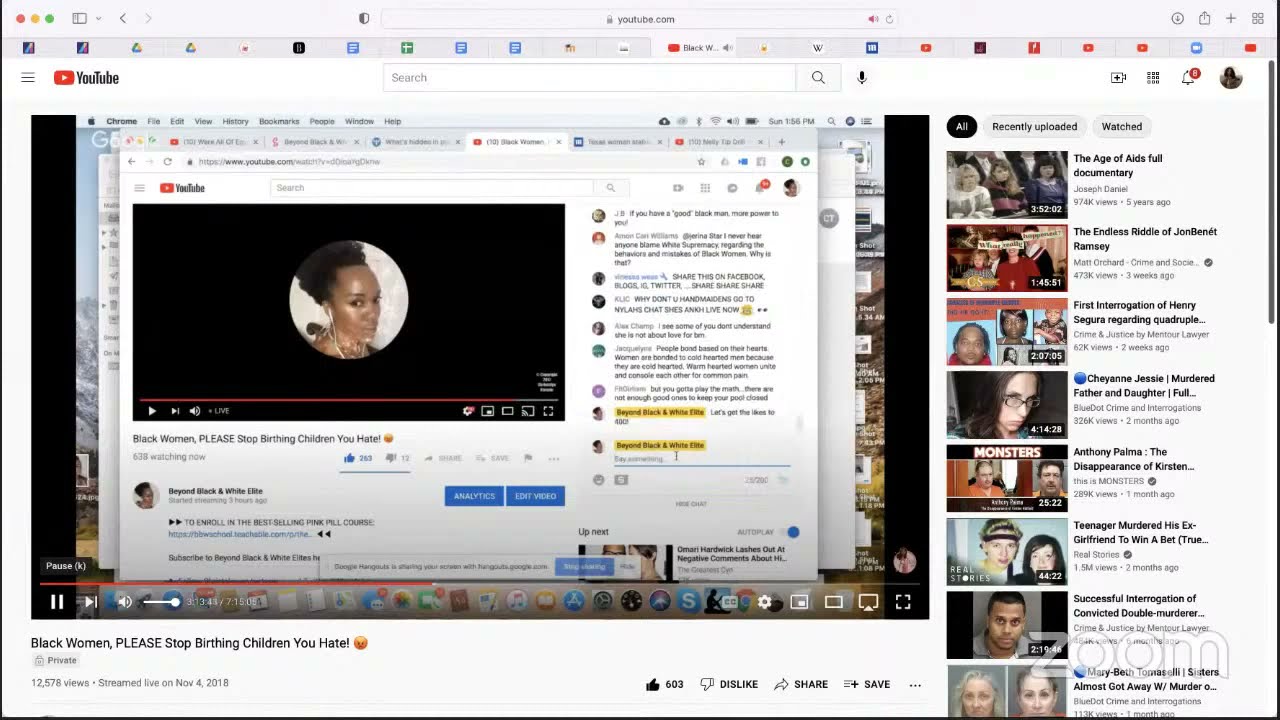The image is a detailed screenshot of a YouTube homepage displayed on a Mac device. The aspect ratio of the image suggests it is about one and a half to two times wider than it is tall. Starting from the upper left corner, we can see the distinctive Mac system buttons—three circles in red, yellow, and green—used for window management. 

Moving right from these buttons, there are additional browser controls, followed by the URL bar displaying "youtube.com," indicating the site is secure with a lock icon to the left of the URL. On the far right of the top bar, there are more icons for various browser functions.

The main area of the YouTube homepage has a white background, consistent with YouTube's standard design. In the upper left, three horizontal lines symbolize the menu, followed by the YouTube logo and the text "YouTube." Centered on the page is a rectangular search bar with a magnifying glass icon to the right and a black microphone icon further to the right.

In the upper right corner are several menu options, including an alerts icon and the user's profile picture, which is dark and shadowed, making it indistinguishable. 

Dominating the main screen is the YouTube video player, which features the usual control buttons at the bottom. These include play/pause, next video, volume controls, and the video progress bar showing the current playback status.